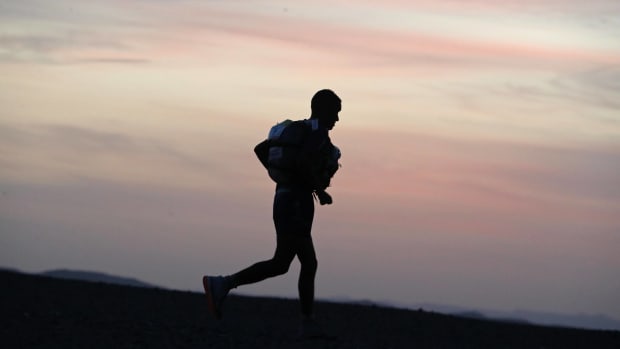The image portrays a male silhouette actively running from left to right against a sky at dusk. The man is entirely black in silhouette, rendering his facial features indistinguishable. His right leg is extended back while his left leg is forward, mid-stride, and his arms mimic a running motion. He appears to be wearing a backpack, suggested by a noticeable bump on his back. The sky behind him displays a blend of colors, predominantly gray with hints of reddish and pinkish tints indicative of either dawn or dusk. The platform he runs on is dark and appears elevated with a slant from higher on the left to lower on the right. In the background, subtle silhouettes of hills and mountains can be discerned, adding depth to the scene.